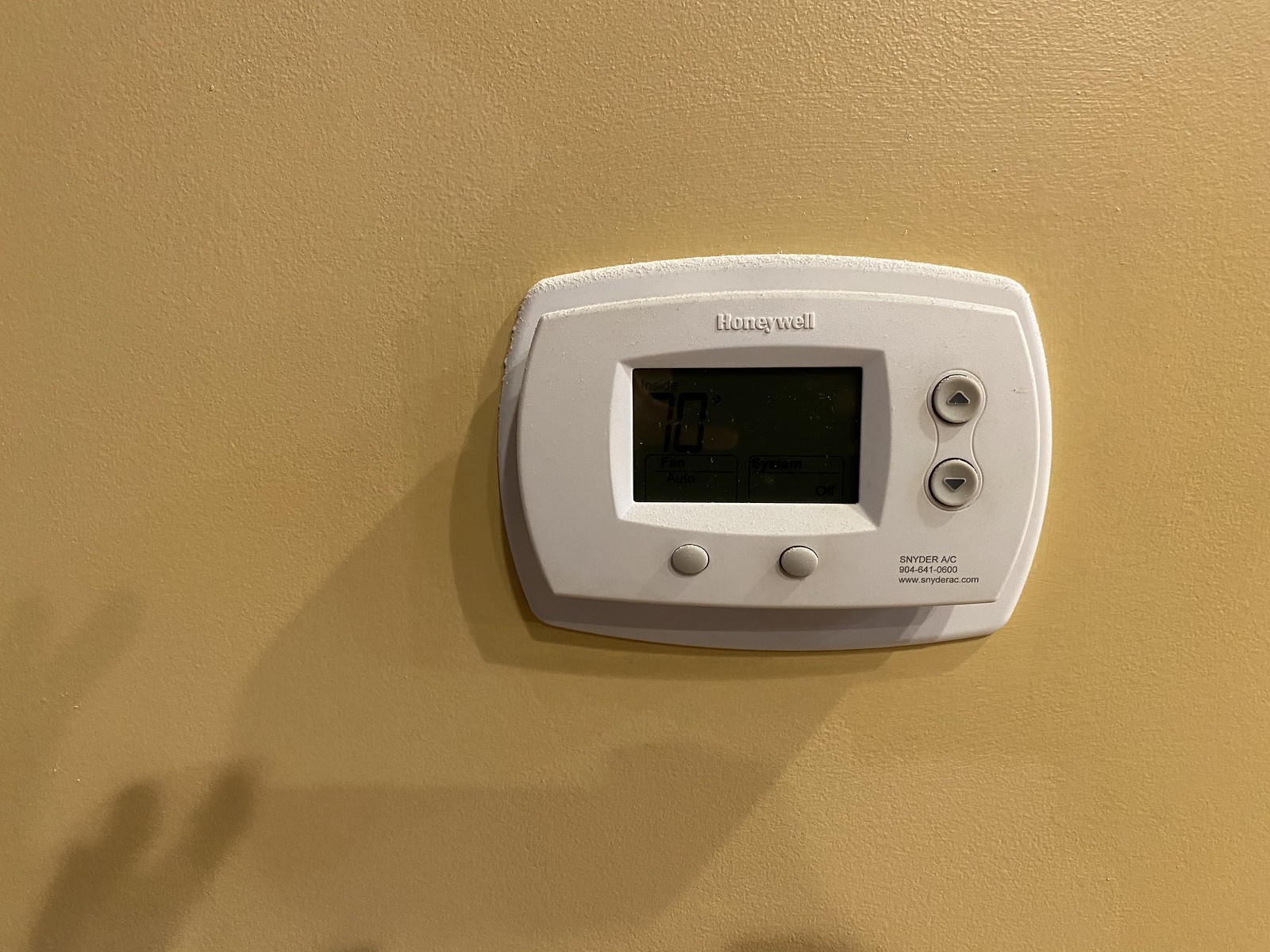The photograph features a Honeywell heating and air conditioning thermostat installed slightly off-center on a wall painted in a rich coffee brown color. The white thermostat prominently displays a somewhat vague temperature reading on its central LCD screen, possibly indicating 70 degrees Fahrenheit. Below the screen, two gray buttons are present, lacking any visible text, presumably for navigation within the device's menu. To the right of the LCD, there are up and down buttons for adjusting settings.

In fine print below the buttons, the label reads "Snyder AC" along with a contact phone number, 904-841-0600, and their website, www.snyderac.com. The wall surrounding the thermostat shows interesting shadow play, likely from two light sources: one directly above or slightly to the right of the thermostat and another from behind the photographer. These shadows form a double image, slightly mysterious and possibly resembling a hand or a staircase rail.